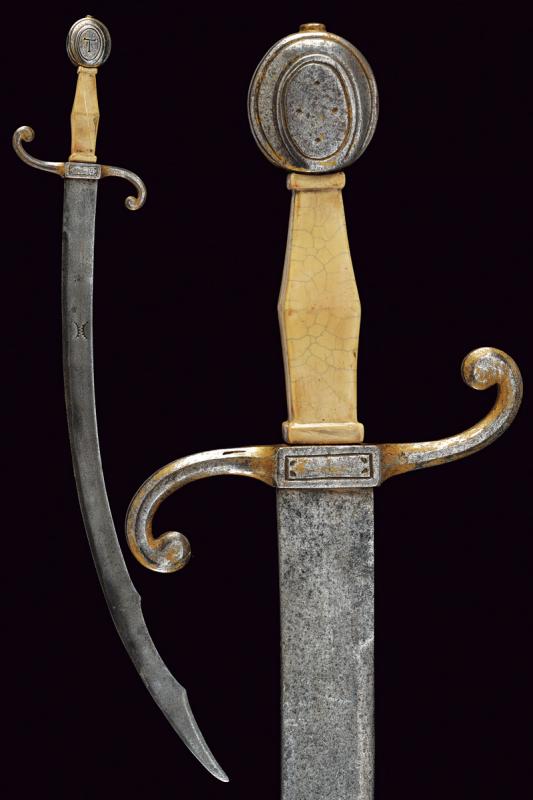This image showcases two views of an antique sword set against a black background. On the left side, the full sword is displayed, featuring a slightly curved, single-edged silver blade with a mix of black patina indicative of its age. The handle is distinctively yellow and extends into a beautifully foiled curvature at the guard, creating a seamless transition from handle to blade. The pommel is oval-shaped and stamped with the letter 'T', while the grip appears to be made of an ivory-like material. On the right side of the image, there is a magnified close-up highlighting the intriguing details of the handle and the guard, echoing the curvature and ornate design seen in the full-length view. The sword, likely hailing from Italy and dating back to the late 15th to early 16th century, has a total length approximating in the low 90 centimeters range.